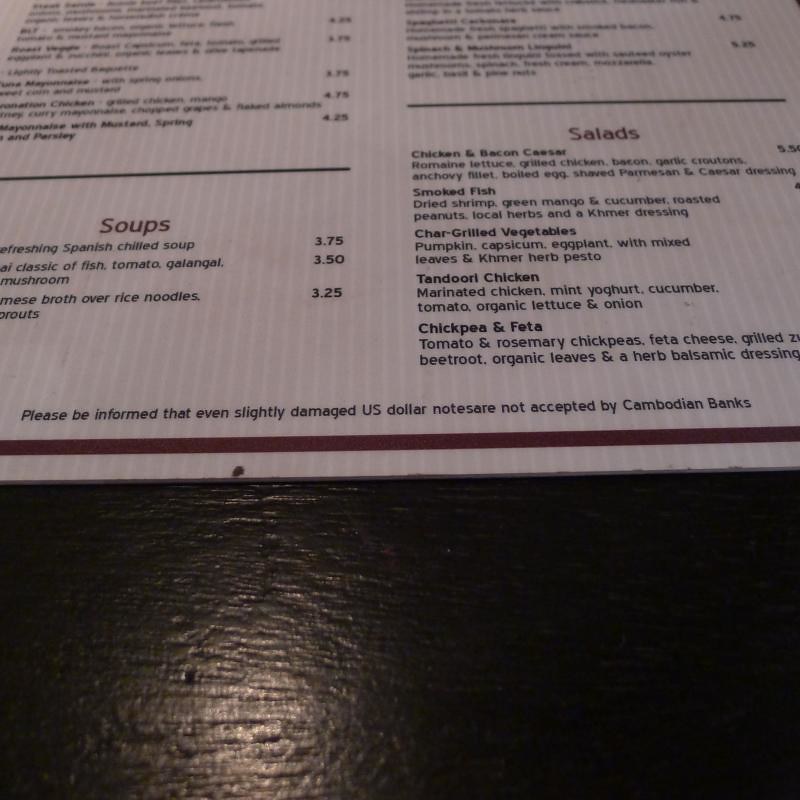This close-up image captures a meticulously detailed section of a restaurant menu, set against the backdrop of a black-painted wooden table, showcasing the subtle wood grain texture. The visible portion of the menu focuses on the soups and salads offered by the restaurant, revealing an interesting and diverse selection. Among the soups, there is a refreshing Spanish chilled soup, a classic soup featuring fish, tomato, galangal, and mushroom, and another with Vietnamese broth poured over rice noodles and sprouts. 

The salads listed are equally varied and enticing, including a chicken and bacon Caesar, a smoked fish salad, char-grilled vegetables, tandoori chicken salad, and a chickpea and feta salad. The detailed description of the chickpea and feta salad mentions specific ingredients such as tomato and rosemary chickpeas, feta cheese, grilled zucchini, beetroot, organic leaves, and an herb balsamic dressing. 

An important note at the bottom of the menu informs patrons that slightly damaged dollar notes are not accepted by Cambodian banks, hinting that this restaurant is likely located in Cambodia and caters to tourists. Additional sections of the menu are visible but not legibly captured in the photograph, suggesting a rich variety of dishes and ingredients throughout.